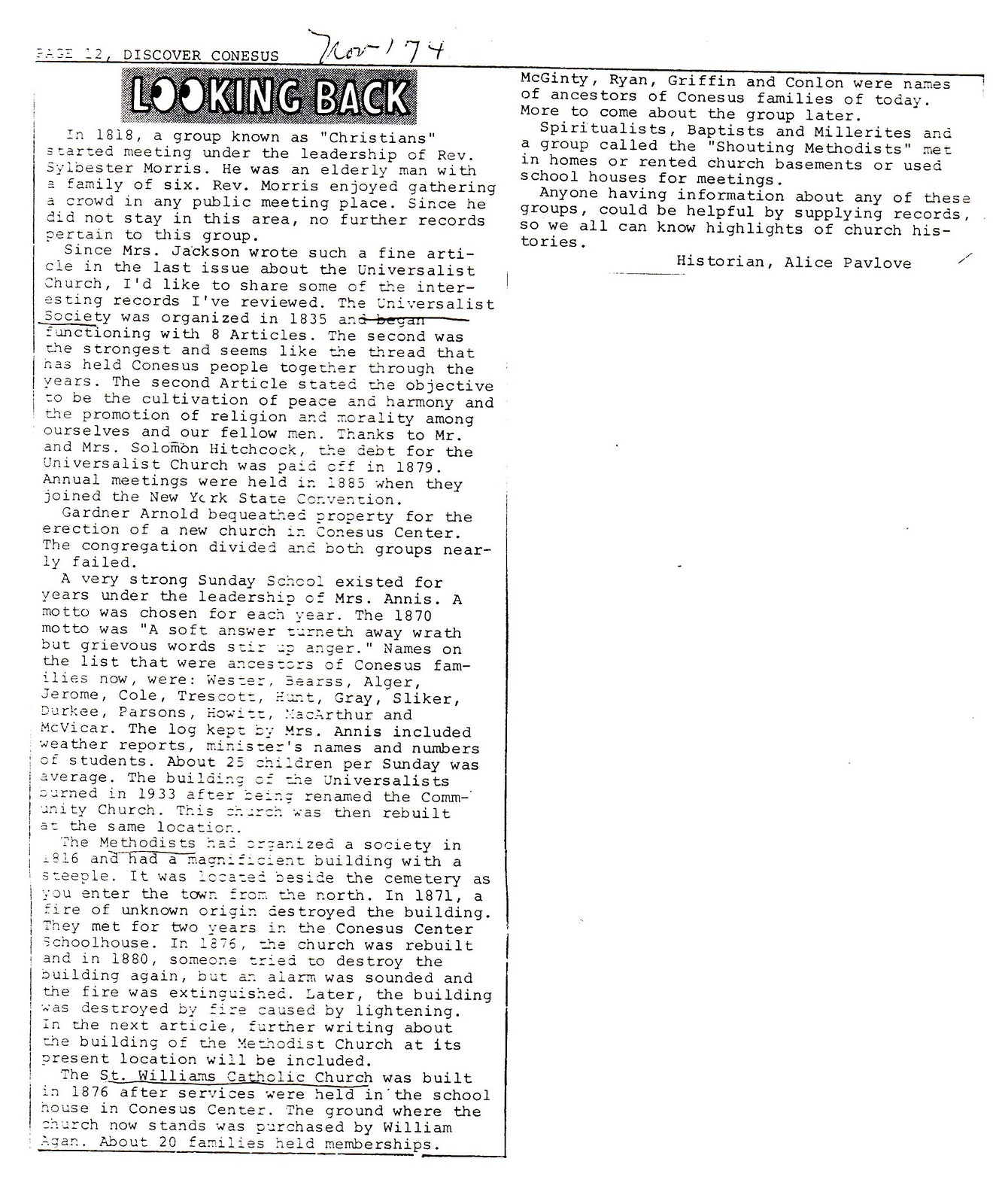This black and white newspaper clipping, dated November 7, 1974, titled "Looking Back" with the O's in "LOOKING" represented by eyeballs, offers a detailed historical account of various religious groups in Conesus. The article, found on page 12 under "Discover Conesus," recounts that in 1818, a group known as the Christians began meeting under the leadership of Reverend Sylvester Morris, an elderly man with a family of six who enjoyed gathering crowds at public meetings. Given that he did not stay in the area, no further records exist about this group.

Following a fine article by Mrs. Jackson on the Universalist church, the piece delves into the 1835 formation of the Universalist Society, noting their objectives of promoting peace, harmony, and moral upliftment. Significant historical events include the 1879 debt repayment by Mr. and Mrs. Solomon Hitchcock and Gardner Arnold's 1885 property bequest for a new church. Names tied to the early Universalist community included Wester, Boris, Alger, Jerome, Cole, among others. The congregation later faced divisions and fires in 1933 and the late 1800s but demonstrated resilience, rebuilding the church each time.

The article then highlights the Methodist society organized in 1916, which also endured fires in 1871 and the late 1870s, leading to multiple reconstructions. Notably, a fire caused by lightning destroyed another iteration of the building. There is mention of the St. William’s Catholic Church, built in 1876 on land purchased by William Alvin, attracting approximately 20 families with surnames like McGinty, Ryan, Griffin, and Conlon.

Brief descriptions of other groups such as Spiritualists, Baptists, Millerites, and Shouting Methodists indicate they often met in homes, rented church basements, or schoolhouses. The article concludes with a call for records to be shared to enrich the collective understanding of Conesus’ church histories, signed by historian Alice Pavlov.